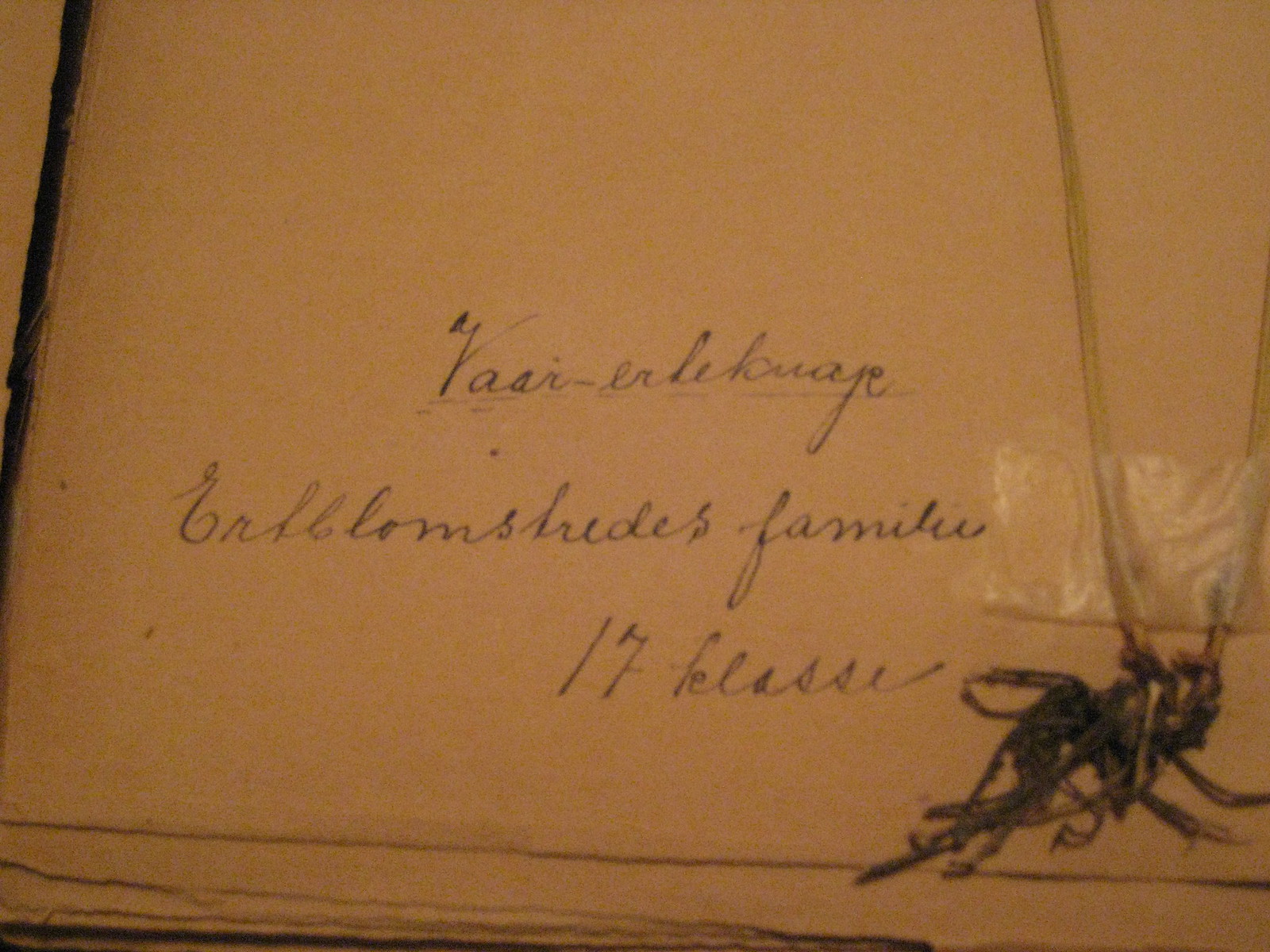The image depicts a very old, weathered page, likely from a scrapbook, journal, diary, or photo album. The paper, an aged ivory with greenish hues, appears rugged and possibly hand-torn, suggesting it may be handmade. This gives the impression of significant antiquity. The scene is dimly lit, adding to the aged and nostalgic atmosphere. On the bottom right-hand corner, a very dead flower or plant has been taped in. The tape, now brownish, secures the black, withered strands of the preserved specimen. To the left of the dead plant, there is some handwritten cursive writing in what seems to be a foreign language, possibly German. Among the scribbles, the number "17" is discernible, while the rest remains unreadable. This intricate collection of elements enhances the sense of historical preservation and personal memory within the image.